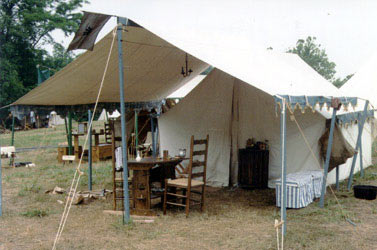The image depicts an outdoor scene set up with a large, white tent featuring silver and blue poles. This tent, supported by light beige ropes, shelters a dining area underneath, complete with a wooden table and chairs. Additionally, there are some coolers under the tent. The ground beneath is a mix of dirt, grass, and patches of greenery, with rich, dark green leaves accentuating the natural backdrop. In the distance, more wooden furniture and possibly other tents are visible, suggesting an arrangement for outdoor dining or a furniture display. The setting appears to be in a sunny, wooded area with trees and foliage surrounding the scene.